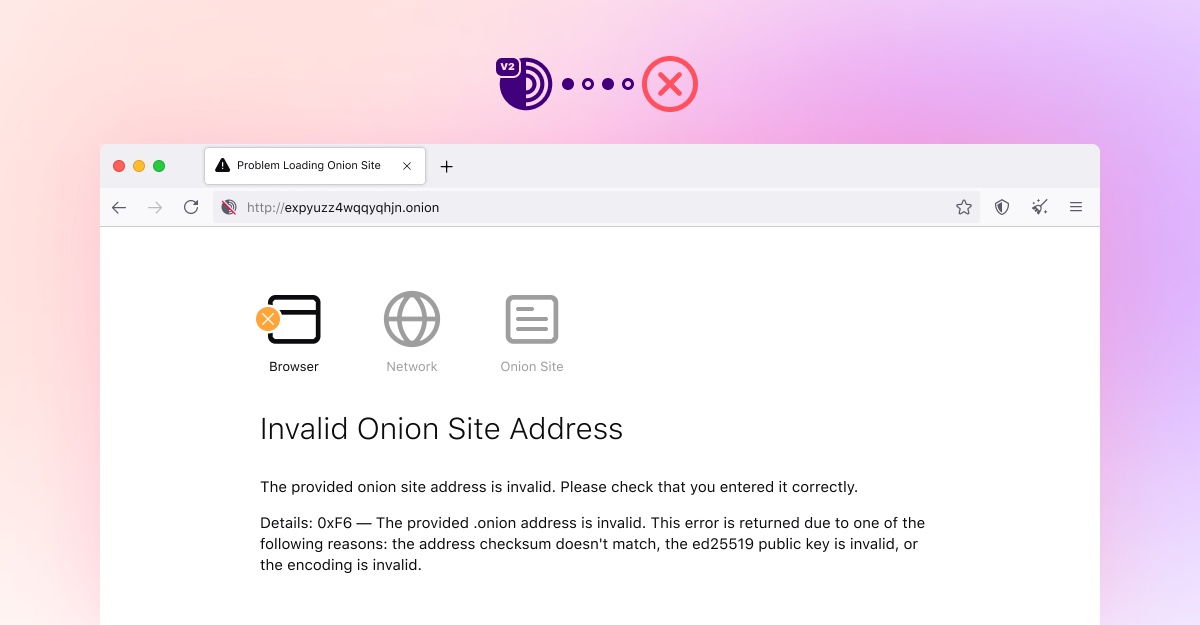The image depicts a web page on a computer screen set against a gradient background of light pink on the right transitioning to peach on the left. At the top center of the page, there is a purple logo with white text that reads "V2." Beside this logo, there are four small circles - alternating between solid and outlined in purple - followed by a red circle with an X inside it. The browser window's tab is labeled "Problem Loading Onion Site," and the address bar displays the URL: "http://expyuzz4wqqyqhjn.onion." Below the address bar, the page displays three icons labeled "Browser," "Network," and "Onion Site." The leftmost icon, representing the browser, is a yellow file icon with an X over it. Beneath these icons is a prominent message stating "Invalid Onion Site Address," accompanied by further details in smaller black text, explaining that the provided Onion address is invalid, likely due to a mismatch in the address checksum or other input errors. This message is on a white background within the browser window, adding to the contrast of the gradient backdrop.